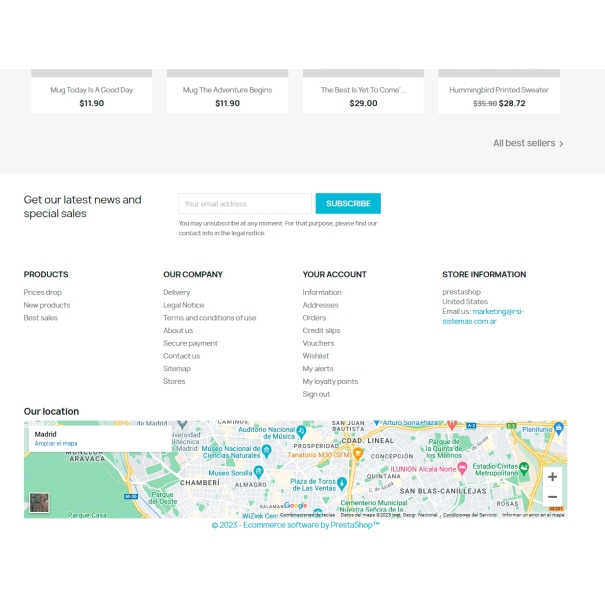The screenshot features a user interface with a light gray horizontal rectangle at the top. Inside this rectangle are four white boxes, each bordered by a thick gray line at the top. Each box contains small black text displaying a price, and on the right, the phrase "All Best Sellers" is visible, accompanied by a right-pointing arrow resembling a sideways V.

Beneath this section is a large white rectangle. On the left side of this rectangle, black text reads, "Get our latest news and special sales." To the right of this text is an outlined rectangle in gray, and further to the right is an aqua-colored "Subscribe" button.

Below are three columns with headings in bold black text: "Products," "Our Company," "Your Account," and "Store Information." Each column has a list of items underneath its respective heading.

At the very bottom is another horizontal rectangle. Above it, on the left side, bold black text states "Our Location," and within this rectangle at the bottom of the screen is an embedded Google Map.